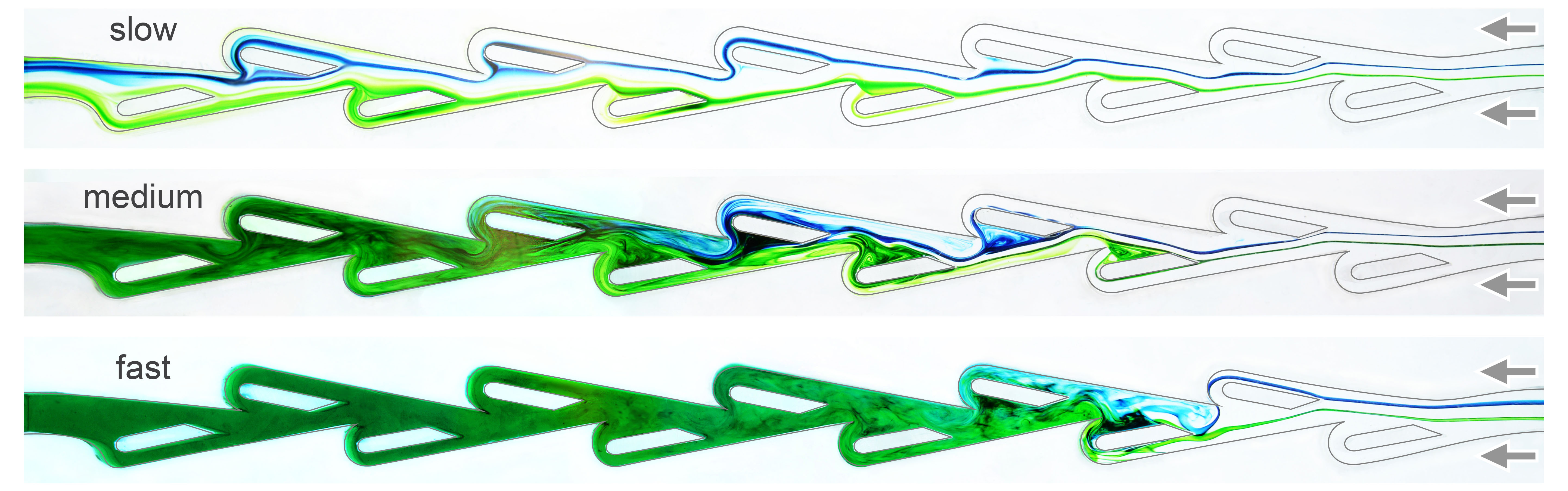This image depicts three horizontally arranged wavy lines, each labeled with one of the words "slow," "medium," and "fast" at the top-left corner in black lettering. The first line at the top, marked "slow," features a subtle flow of light green and blue colors. The second line in the middle, labeled "medium," shows a more pronounced green with a slight presence of blue. The third and bottom line, labeled "fast," displays a dominant and uniform shade of green with only a faint touch of very light blue. The lines, reminiscent of zigzag patterns or tubes with handles, are ordered vertically, one below the other, and have sections protruding upwards and downwards along their paths. The right side of the image includes two leftward-pointing arrows, further emphasizing the progression from slow to fast.